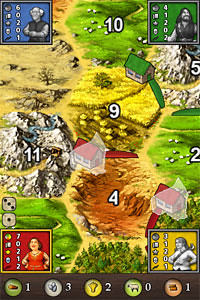The image appears to be a detailed rendering, likely a screenshot from a mobile video game, showcasing an overhead view of a diverse landscape. The map includes a myriad of terrains such as green grasslands, a yellow-hued valley that could be composed of sand or rock, white-capped mountains, and sections of lush green areas. There are notable structures, including two red-roofed houses, a green-roofed house, and what seems to be two red bridges spanning across the orange valley.

In each of the four corners of the image, there are character portraits framed by colored backgrounds, each accompanied by various numerical values and icons. The top left corner features a blue background with an older, bald man having white hair on the sides. This image is labeled with numbers, including 60201, and features several icons with different items and their respective quantities. The top right corner showcases a man with a beard and longer hair set against a green background, also accompanied by several numerical indicators. The bottom left corner depicts a woman in a red dress, standing confidently with her hands on her hips, framed by a red background and noted with various numbers. Finally, the bottom right corner displays a woman dressed in white, set against a yellow background and marked with additional numerical figures.

Additionally, the map contains designated numbered regions such as a grassy area labeled 10, a yellow field labeled 9, mountain terrain marked as 11, a brown region labeled 4, and another green area marked 2, adding further detail to the intricacies of the landscape depicted in the image.